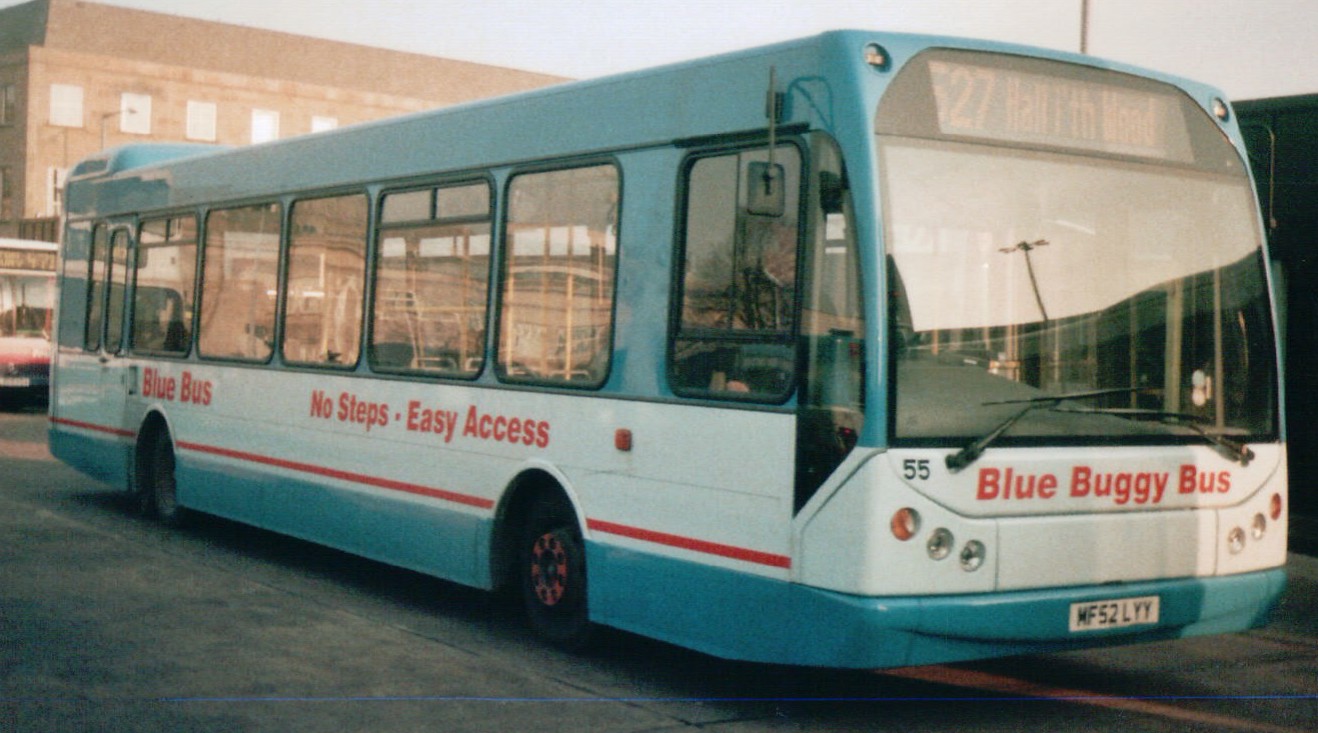The image depicts a detailed street scene in a landscape orientation, showcasing a single-story blue-decked bus parked at a curb on a road. The bus, taking up most of the foreground, features a light blue roof and large, clear windows. A wide white stripe bisects the middle of the bus horizontally, with an additional narrower blue stripe below it and a red stripe above it. Bold red text on the side announces, "Blue Bus, No Steps, Easy Access". The front of the bus displays "Blue Buggy Bus" in orange lettering, flanked by three headlights on each side and a large windshield with visible wipers. Above the windshield, a digital display reads "527", presumably indicating the route. An ID plate marked "MF52LYY" is also visible on the bus' front. Behind this bus, there is another parked bus and a two-story brick building, all set against a clear blue sky.